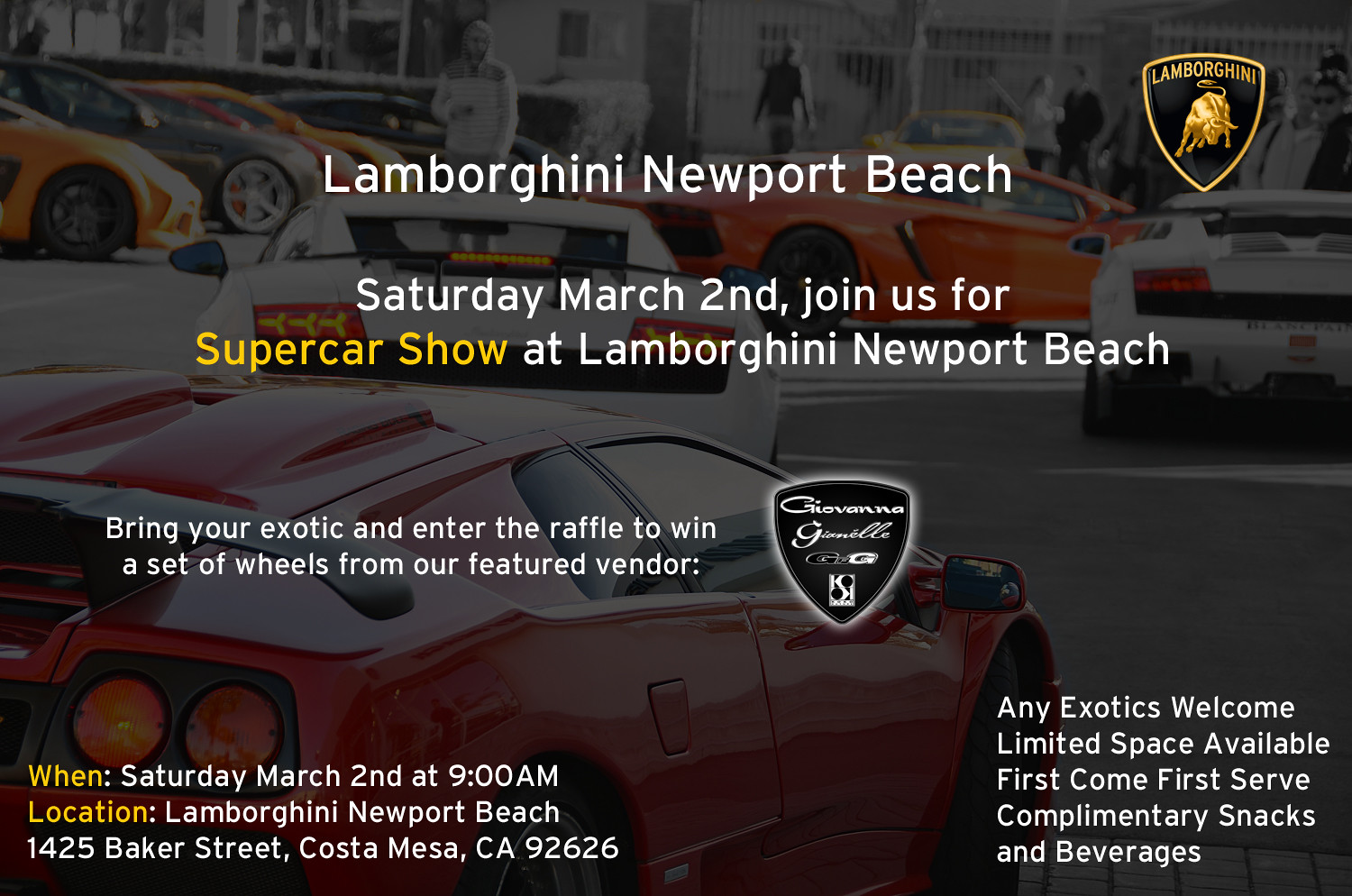The image is an infographic advertisement for a supercar show held at Lamborghini Newport Beach. The event took place on Saturday, March 2nd at 9 a.m. at 1425 Baker Street, Costa Mesa, California, right next to Newport Beach. The background features several Lamborghini cars in various colors—red, white, and orange—either parked or driving, with the image slightly dimmed to make the overlaid text stand out. 

The Lamborghini logo, a black shield with a golden bull, is positioned in the top right corner. The main text reads, "Lamborghini Newport Beach, Saturday, March 2nd. Join us for a supercar show at Lamborghini Newport Beach." The text emphasizes that any exotic cars, not just Lamborghinis but also marques like Aston Martin and Porsche, are welcome. 

The event offers limited space on a first-come, first-served basis, with complimentary snacks and beverages available. Additionally, attendees can enter a raffle to win a set of wheels from the featured vendor, Giovanna Gianelli. The promotional text uses gold for "supercar show" and white for the other information, designed to stand out on a social media platform.